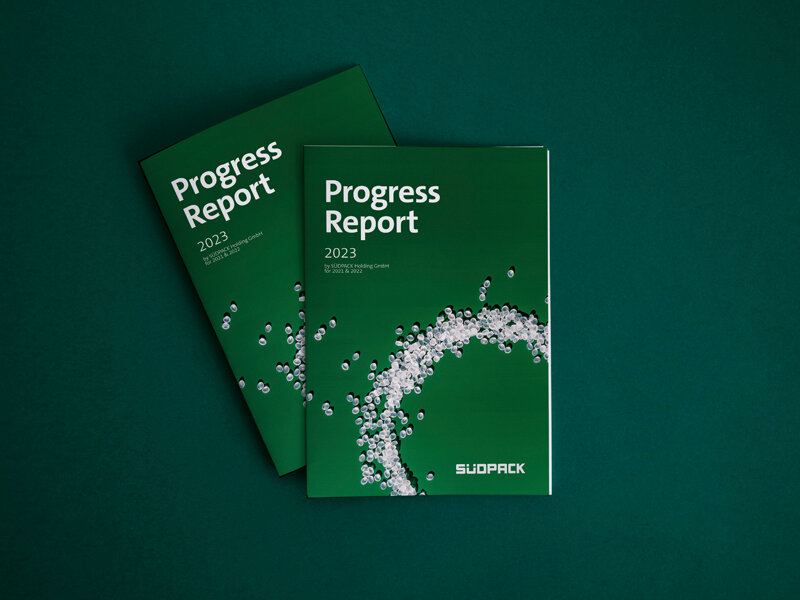In the image, there are two identical, green pamphlets with white text, layered one on top of the other, slightly tilted to the left. The pamphlet on the bottom is partially visible and both have "Progress Report 2023" written prominently on the top with some smaller, unreadable text below. Just above the bottom edge of the pamphlets, the brand name "SUDPACK" is printed. An eye-catching feature is a half-circle arc of crystal-like beads stacked together, appearing to form a dazzling array stretching from the bottom to the middle of the pamphlets. The pamphlets are set against a dark green backdrop, casting deep shadows to the upper left. Tiny slivers of the white pages inside the pamphlets are visible along the right edge and the top strip of the lower booklet. The overall color palette of the image includes varying shades of green and white, lending it a harmonious and striking appearance.